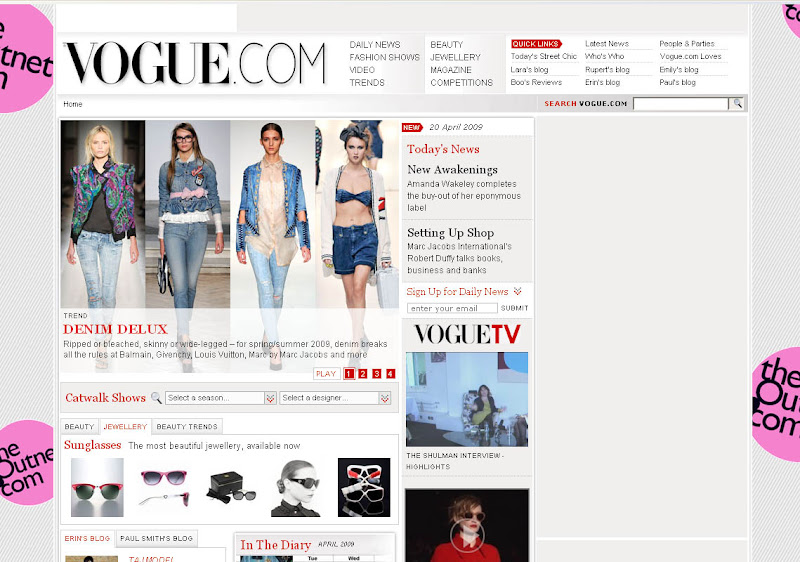The webpage from Vogue.com presents a well-organized and visually appealing interface. At the top left corner, the bold black text reads 'Vogue.com', followed by a series of navigation tabs on the right, including 'Daily News', 'Fashion Shows', 'Videos', and 'Trends'. Additional tabs on the far right include 'Beauty', 'Jewelry', 'Magazine', and 'Competitions'. 

The quick links, located in the top corners, feature 'Today's Street Check', 'Lara's Blog', 'Bulls Reviews', 'Latest News', 'Who's Who', 'Rupert's Blog', 'Erin's Blog', 'People and Party's Vogue.com', 'Love's', 'Emily's Blog', and 'Paul's Blog'. Directly below these links is a search bar with the prompt 'Search Vogue.com'.

On the left side of the page, four models are displayed under the headline 'Trend: Deluxe Denim'. The text underneath reads, "Ripped or Bleached, Skinny or Wide-Legged for Spring or Summer 2009, Denim breaks all the rules at Balmain, Givenchy, Louis Vuitton, Marc by Marc Jacobs, and more."

The lower section features 'Beauty' and 'Jewelry' categories, with 'Jewelry' highlighted in red, indicating it as the selected category. Below it, a collection of five pairs of sunglasses is showcased, with a description that reads, "Sunglasses are the most beautiful jewelry available now."

On the right side of the page, the 'Today's News' section highlights 'New Awakening', mentioning Amanda Wakeley who completes the Beauty out of Hair eponymous label and has a segment titled 'Selling Up Shop'. Finally, there's an option to 'Sign Up for Daily News' at the bottom.